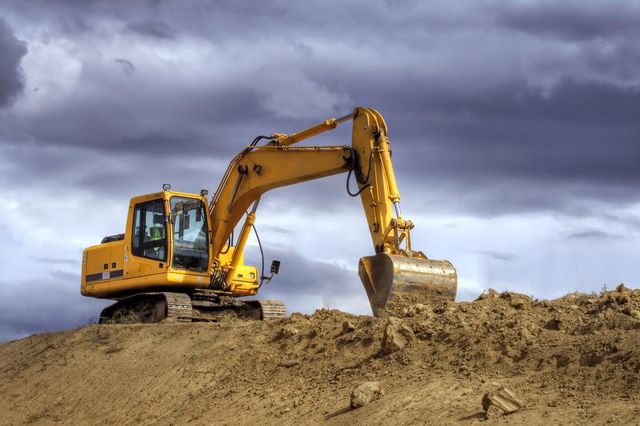The image captures a yellow piece of heavy construction machinery that appears to be a bulldozer, excavator, or backhoe. This machine, equipped with a large metal scoop or bucket and metal tracks for movement, is positioned prominently atop a mound of brown, solid dirt. The scoop is extended, engaged in digging or preparing to scoop up the loose soil on the hill. The scene is set against a dramatic, dark sky filled with stormy clouds, hinting at an approaching storm. The background shows no clear sky, only an expanse of ominous gray clouds. There appear to be dirt and rocks scattered around the excavation site. Despite some ambiguity, it seems there might be a person inside the machine’s glass cab, though it's not clearly visible. The overall scene gives an impression of intense labor under impending stormy conditions.